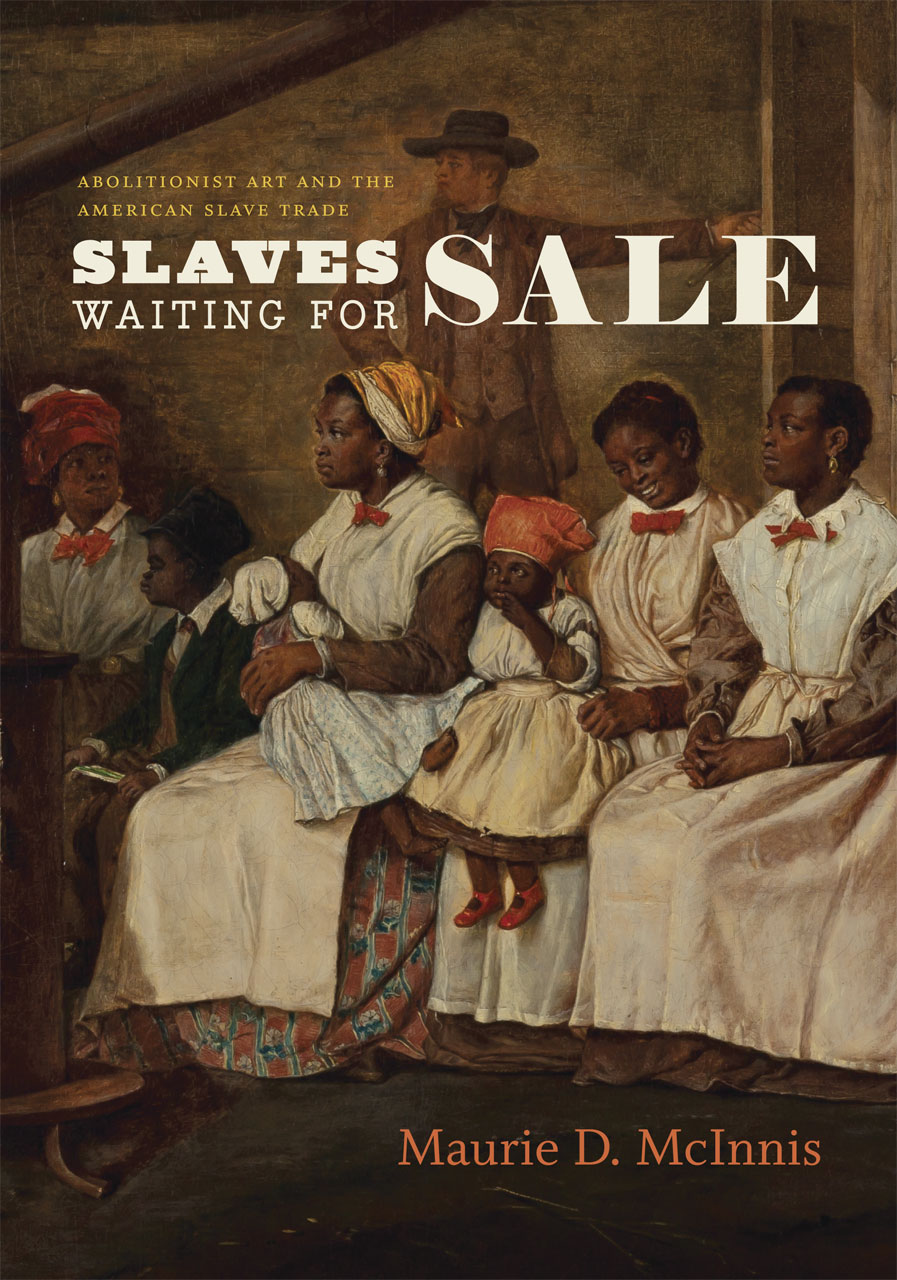The image appears to be the detailed cover of a book titled "Abolitionist Art and the American Slave Trade," presented in yellow font. Dominating the cover is a poignant drawing of six African Americans, likely slaves, consisting of four women, two children, and a baby. The women are adorned in printed or brown dresses paired with white aprons, some highlighted with small bows around their necks. One of the children, a little boy, is dressed in a suit and hat. Another child, a girl, parallels the women's attire but distinguishes herself with red shoes and a red scarf. The baby is depicted in a white dress and hat but is shoeless. Overlooking this sorrowful group is a white man in a dark suit and hat, standing to the rear and appearing somewhat disengaged. The title "Slaves Waiting for Sale" is prominently displayed in bold white letters, and the author's name, Maurie D. McInnis, is inscribed at the bottom in white font. The background is predominantly dark, with grayish tones enhancing the somber mood of the artwork.